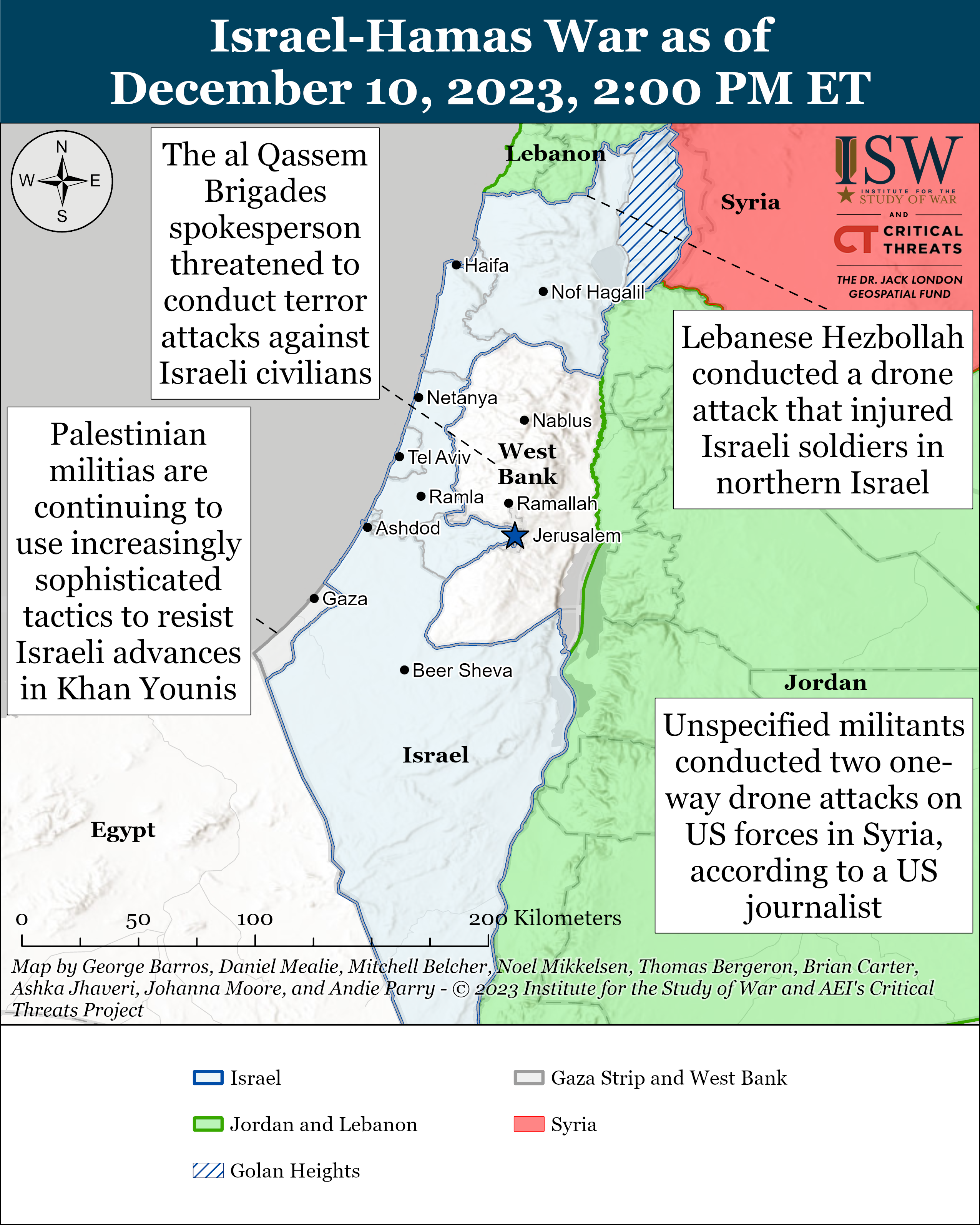The image is a detailed map highlighting the geopolitical situation involving Israel, Egypt, Jordan, Syria, and Lebanon, updated as of December 10, 2023, at 2 p.m. ET. At the top, a headline in a blue stripe reads, "Israel-Hamas War as of December 10, 2023, 2 p.m. ET." Israel is prominently featured in the center, shaded in blue, with the West Bank marked in white. To the right of Israel, Syria is colored red, and a text box notes: "Unspecified militants conducted two one-way drone attacks on U.S. forces in Syria according to a U.S. journalist." Lebanon is located to the north of Israel, shaded in green, with a text box indicating that "Lebanese Hezbollah conducted a drone attack that injured Israeli soldiers in northern Israel."

To the southwest of Israel, Egypt is visible, and at the bottom, there's a ruler measuring distances from 0 to 200 kilometers. A compass rose is positioned in the left-hand corner of the map for orientation. There are several text boxes providing updates: one in the upper left notes the Al-Qassam Brigade spokesperson's threat to conduct terror attacks against Israeli civilians, another states Palestinian militias are using sophisticated tactics against Israeli forces in Khan Younis.

The key at the bottom of the image clarifies the color coding: blue for Israel, green for Jordan and Lebanon, white stripes for the Golan Heights, white for Gaza Strip and West Bank, and red for Syria. Credits for the map's creation are also listed at the bottom, alongside the key.